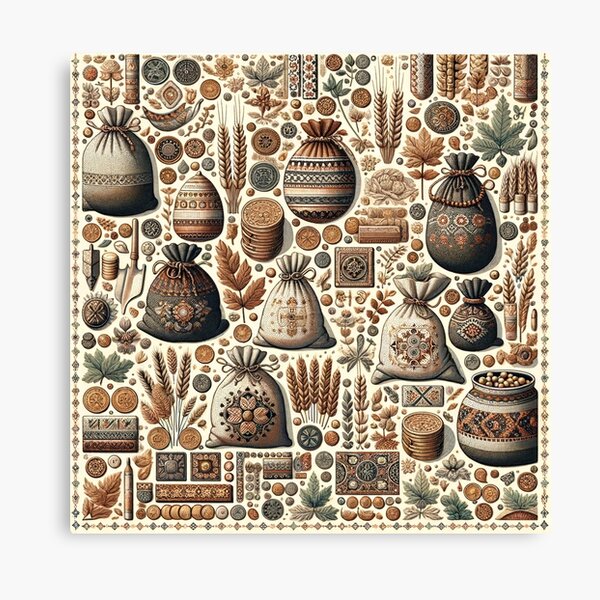This detailed art print on a light yellow background features an intricate and densely packed arrangement of natural and everyday objects. Predominantly, oval, bell, and vase-shaped items are depicted in abundant quantities across the composition. The lower portion of the image is adorned with brown leaves and a series of round shapes transitioning in shades from brown to gray and back to brown. Adjacent to this, a cylinder with a nozzle is visible, coupled with a circle embellished with black indentations around the inner part. Additional brown and gray leaves appear towards the right side.

The mid to upper section of the image includes a collection of vase or bell-shaped objects shaded in gray-brown, alongside a gray-bottom jar containing round balls. The top right highlights a small vase holding chaffs of wheat. In the very top-center, light brown and beige cylinders extend vertically.

The upper left introduces a vertical array of circles alternating in hues of gray and brown. Throughout the image, various bags – reminiscent of burlap bags – and vessels, some filled with grains or depicting food, break the uniformity of the natural motifs. Decorative elements such as black-floral patterns, triangularly edged bags, and an edging pattern frame the entire artwork, contributing to its decorative and elaborate aesthetic. The overall visual impression is that of an artful collage, rich in texture and repetitive natural themes, akin to an intricate wallpaper design.